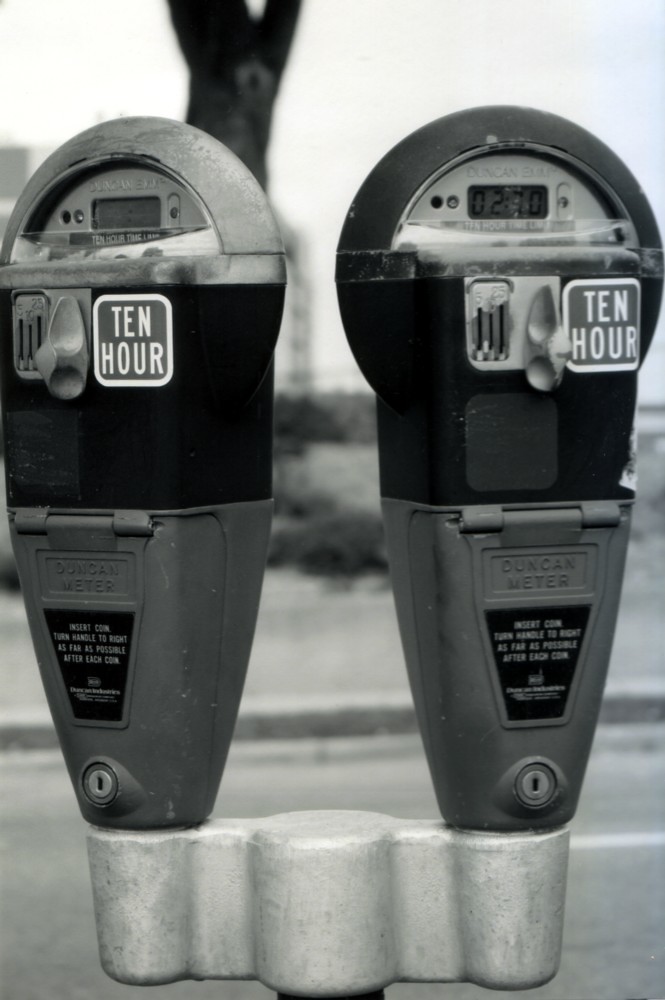This black-and-white photograph captures two slightly aged parking meters standing side by side, attached to a shared metallic base that forms a T-shape, with each meter branching out in opposite directions. Despite the overall dated appearance of the image, the meters are equipped with digital time displays, a modern touch that contrasts with their otherwise vintage design. Each meter features distinct sections: a triangular gray lower portion that converges to accommodate a coin slot, a dial for adjusting time, and a keyhole for maintenance. Above this, a black, box-like section prominently displays a "10 hour" sticker. The uppermost part of each meter, semi-circular in shape, contains the digital readout, with the left meter showing no time and the right meter displaying 2:30. The background is blurred, hinting at a street with a parking spot in front of the meters, while the meters themselves bear the "Duncan" logo and operational instructions for inserting a coin and turning the handle.